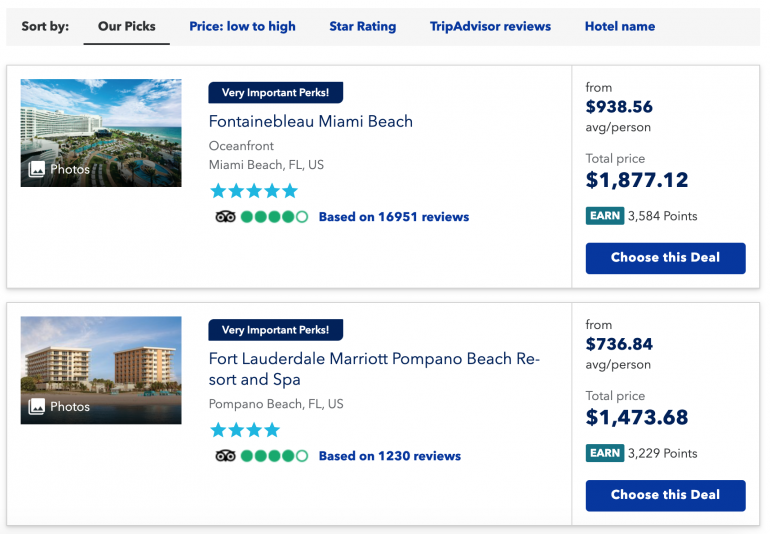**Detailed Descriptive Caption:**

On a TripAdvisor travel booking site, the main menu at the top features various sorting options, including "RPICS" which is underlined in black, indicating it is the currently selected choice. The other sorting options—"price low to high," "star rating," "TripAdvisor reviews," and "hotel name"—are presented in blue text.

Displayed are two resort options, each housed in white fields with thin gray borders.

1. **Fontainebleau Miami Beach:**
   - An image showcases the luxurious Fontainebleau Miami Beach with the scenic ocean on the left and the hotel prominently featured.
   - A blue tab on the right highlights "Very Important Perks."
   - Below, the hotel is described as oceanfront, located in Miami Beach, Florida, USA, and is rated five stars in light blue text.
   - The TripAdvisor logo (an owl) indicates a rating of four out of five circles, based on 16,951 reviews.
   - Pricing details state an average cost of $938.56 per person, with a total price of $1,877.12.
   - Visitors can earn 3,584 points by choosing this deal, with a clear option to "Choose this deal" provided.

2. **Fort Lauderdale Marriott Pompano Beach Resort and Spa:**
   - The displayed image features the hotel's two towers against a coastal backdrop.
   - The property is labeled as Pompano Beach, with a four-star rating denoted by four out of five circles, based on 1,230 reviews.
   - The average price is listed at $736.84 per person, resulting in a total of $1,474.68.
   - Selecting this deal allows guests to earn 3,229 points, again with an option to "Choose this deal" readily accessible.